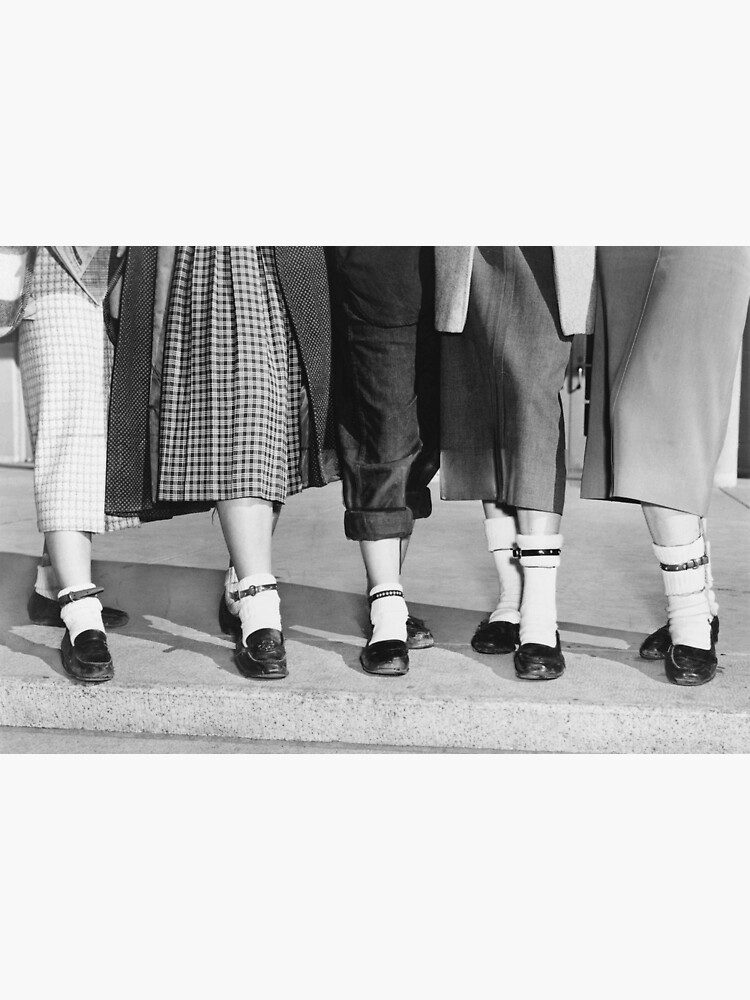This black-and-white photo captures the lower halves of five women standing on a light-colored sidewalk, bordered by a light gray curb that runs from the bottom left to the right edge of the image. Each woman is wearing black slip-on leather shoes paired with white socks. The three women on the left sport shorter ankle-length socks, while the two on the right have taller socks reaching mid-calf, all adorned with a small black belt-like strap around the top. Their outfits are a striking mix of skirts and one pair of pants, reflecting a vintage, possibly 1950s aesthetic. Going from left to right, the first woman wears a light-colored polka-dotted skirt, the second has a darker polka-dotted skirt combined with a cardigan, the third, situated in the center, is distinct with rolled-up black denim pants. The fourth woman dons a dark gray skirt, and the fifth, on the far right, wears a lighter gray skirt without any design. The women's attire, particularly their long skirts and stockings, adds a nostalgic charm to the photograph.